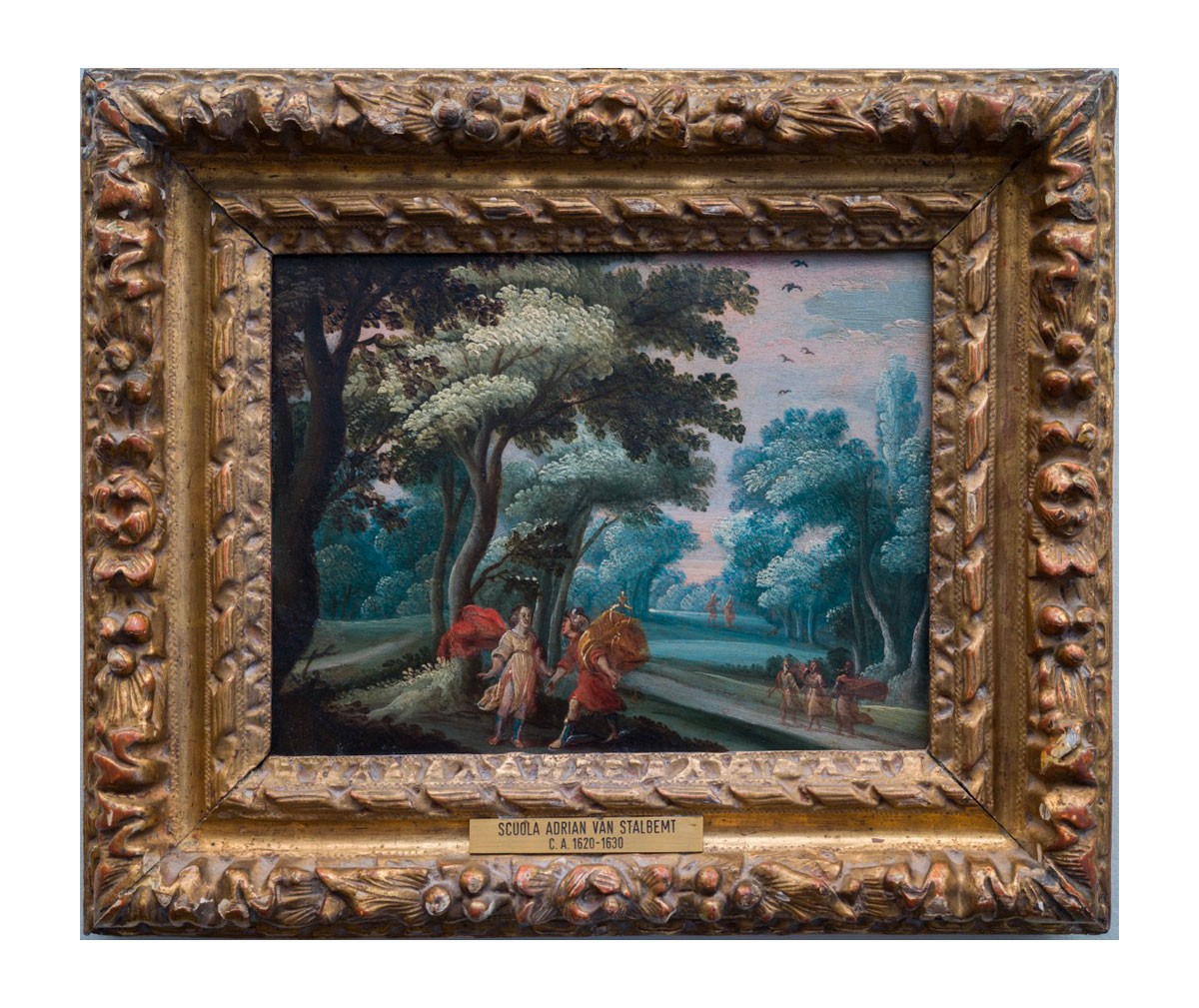This is a color image of an old, ornately carved wooden frame surrounding a small, likely oil painting, marked with a gold nameplate that reads, "Scuola Adrian van Stalbendt, c.a. 1620-1630." The painting, with its vibrant and primarily greenish palette, depicts an outdoor evening scene in a Renaissance realism style. In the center, a man and a woman, dressed in flowing garments with shoes that strap up their legs, appear to be greeting each other, their clothes blowing in the wind. To their right, three figures, presumably women, walk towards the couple, while two additional figures are seen in the distant background among tall trees colored in hues of blue, green, and gray. The top right corner of the painting features a partly cloudy sky with five birds flying in a classic V formation. The thick, layered gold frame adds grandeur to the piece, making it appear larger than it is.